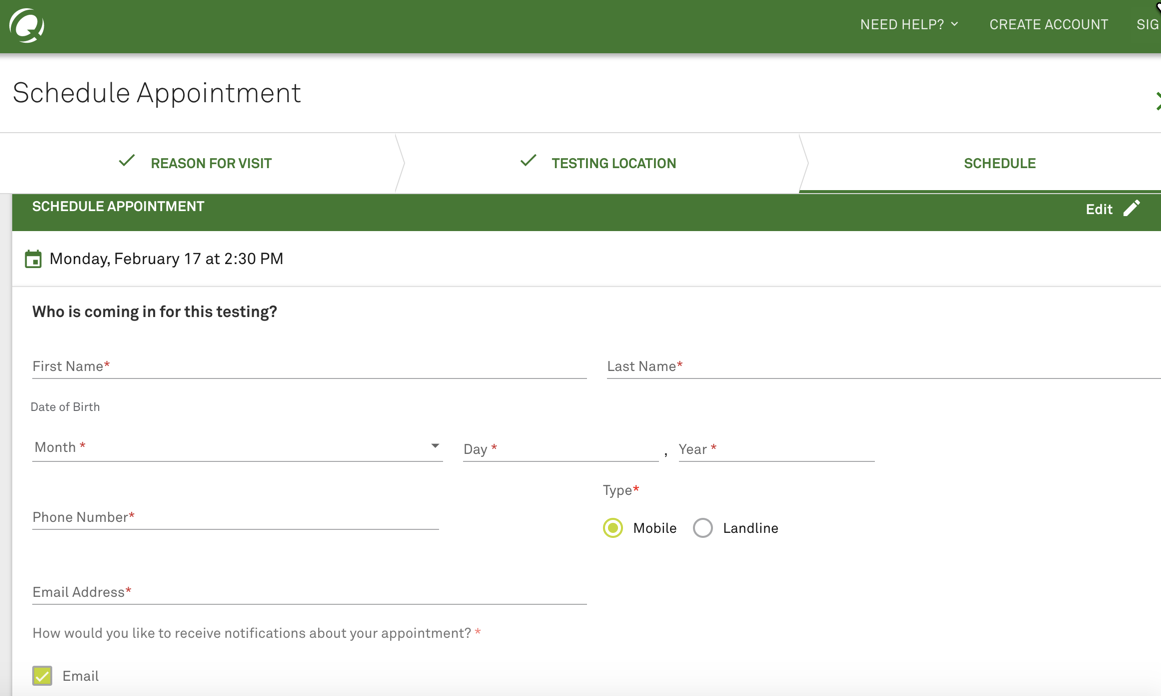A detailed depiction of the scheduling interface is as follows:

The interface's top section features a dark green border. Located in the upper right corner, the options "Need Help," "Create Account," and "Sign In" are prominently displayed. Below this, the main section of the page has a white background with sections designed for scheduling appointments. 

First, there is a button labeled "Schedule Appointment." Underneath, green checkmarks indicate completed sections: "Reason for Visit" and "Testing Location." To the right of these, there is an option to proceed with "Schedule."

Moving further down, another green box is divided into two parts - the left side reads "Schedule Appointment" while the right side shows an "Edit" option, identifiable by a pencil icon. Below this section, the interface switches back to a white background, displaying the scheduled date: "Monday, February 17th at 2:30 p.m."

Following the date and time, there is a query: "Who is coming in for this testing?" Beneath this, fields are provided for "First Name" and "Last Name," followed by sections for the "Date of Birth" comprised of individual boxes for the month, day, and year. 

Further down, contact information fields are presented. On the left, a field for "Phone Number" is available, while on the right, there is a "Type" selection with two circle options: one for "Mobile" and one for "Landline," with the "Mobile" option pre-selected. Finally, the section concludes with a field for "Email Address."